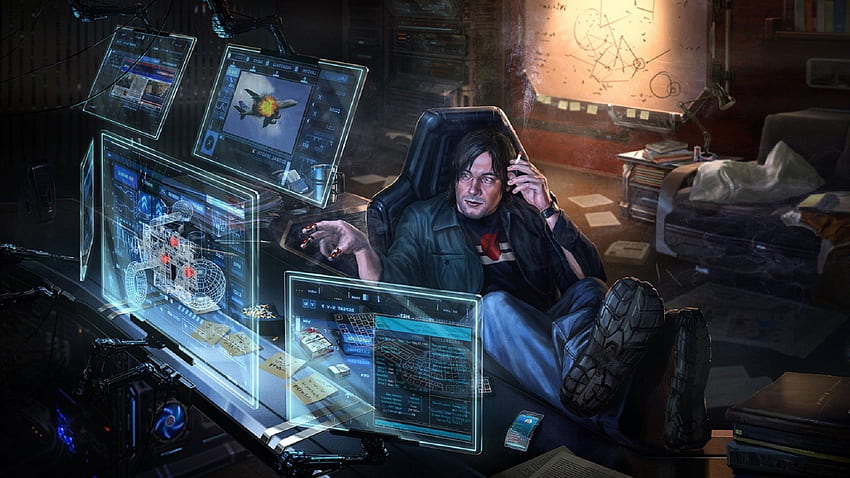In this detailed digital illustration, a disheveled man sits in a plush gaming chair, immersed in a futuristic workspace. Dressed casually in a t-shirt, unbuttoned button-up shirt, jeans, and sporty shoes, he looks weary, sporting a five o'clock shadow and a cigarette in his right hand. His left hand is adorned with rings on his fingers, possibly used for controlling his holographic computer setup. The workspace is cluttered with stacks of paperwork and books, hinting at a lengthy, intense work session. Translucent screens form a semi-circle in front of him: a central large screen, flanked by two medium screens at the top angled downward, and two additional screens on either side angled toward the center. Behind him, a whiteboard or large piece of paper covered in geometric drawings and scribbled notes is visible under a glaring light, adding to the chaotic, yet intensely focused atmosphere. The scene evokes a vibe reminiscent of a young Tony Stark, entrenched deeply in his high-tech, yet cluttered, creative environment.